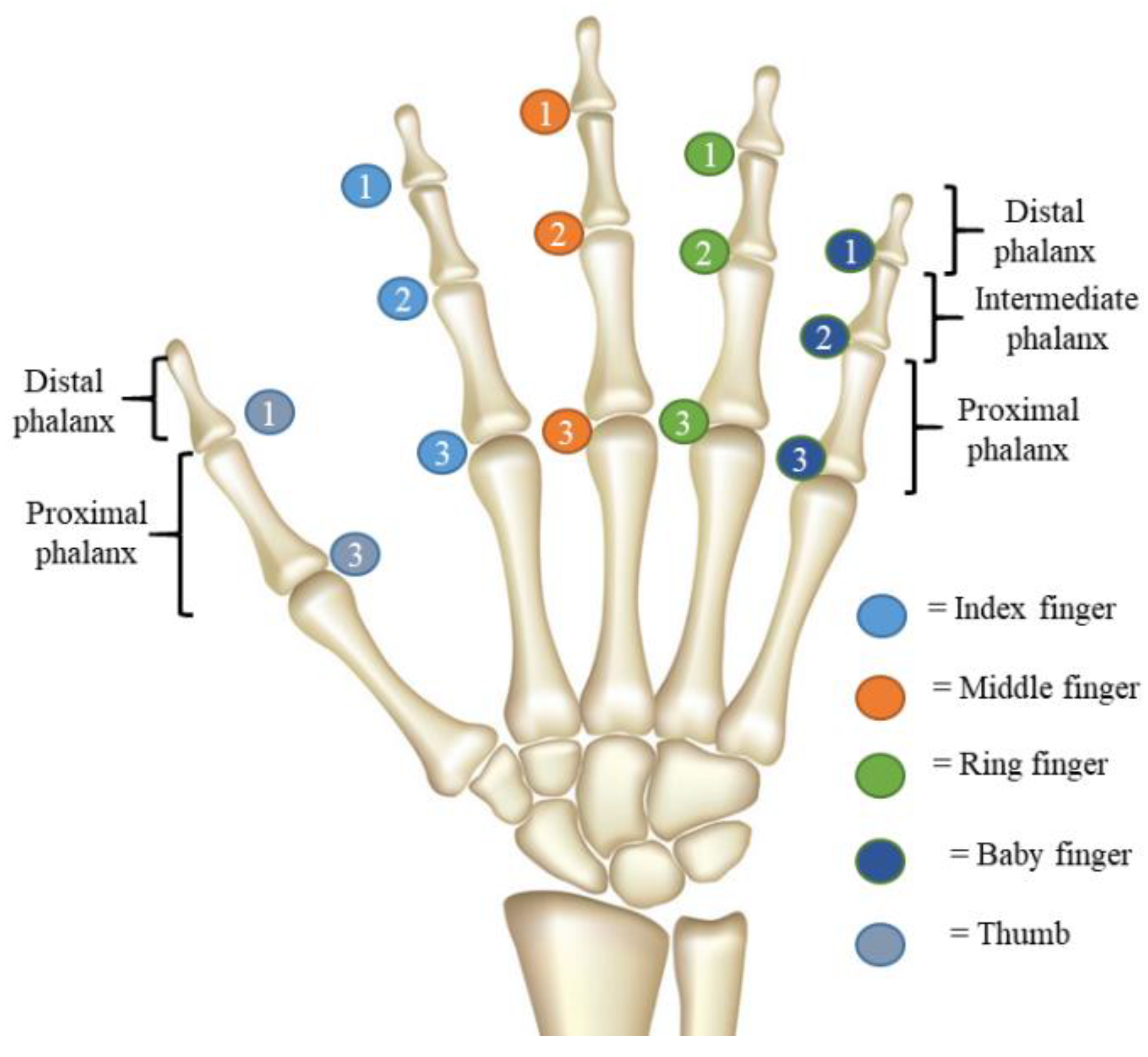This detailed diagram of a human hand's skeletal structure meticulously labels the various bones using a combination of color-coded sections and a numerical key. The bones are depicted in a cream color and the diagram is annotated with terms such as distal phalanx, intermediate phalanx, and proximal phalanx located both on the left-hand side and the top-right corner of the image. Each section of the hand is identified according to the specific part of the finger, including the index finger, middle finger, ring finger, baby finger, and thumb. These sections are distinguished by different colors: blue for the index finger, orange for the middle finger, green for the ring finger, dark blue for the baby finger, and gray for the thumb. A key in the bottom right-hand corner provides corresponding numbers to shades of blue, green, and orange, helping to identify each specific bone's location within the hand. The diagram is likely a textbook extract, noted for its precise and educational illustration of hand anatomy.